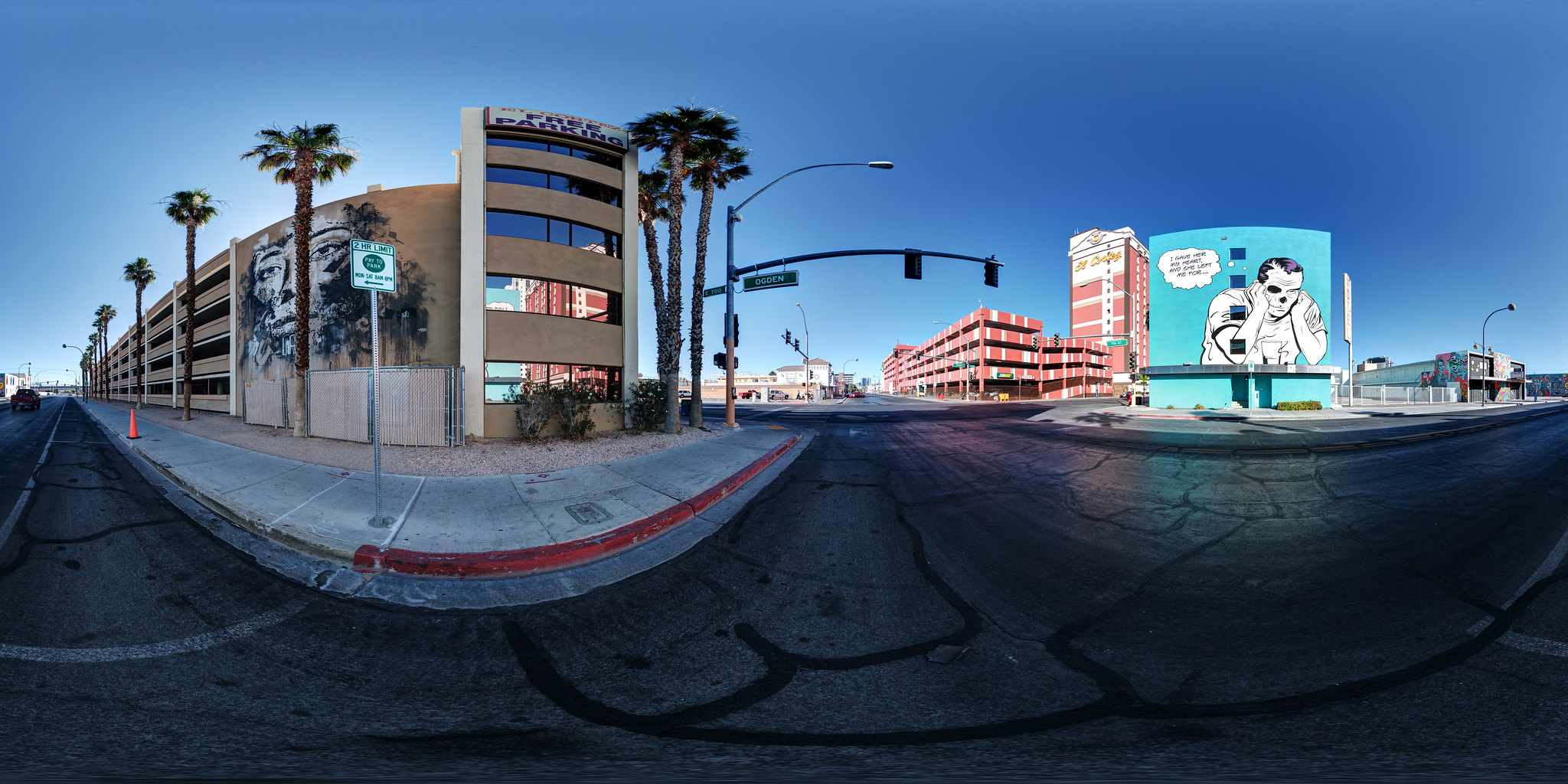The digital photograph captures an outdoor scene, seemingly taken with a fisheye lens that lends a distinctive curvature to the image. The upper left part of the photograph features a baby blue sky, completely clear of clouds, which gradually shifts to a darker blue as you move towards the right. The scene is set at an intersection corner where black asphalt roads are prominently visible. The roads are marked with dark patches where cracks have been meticulously filled in with a deep black material. Faint line markings are also apparent on the left side of the road. A black vehicle is situated on the left, though its direction of movement is ambiguous.

On the left side of the photograph, a gray concrete sidewalk bordered in red—likely indicating a fire lane—runs parallel to the road. Towering palm trees with thick, brown trunks and lush green fronds line the edge of the sidewalk. Behind the row of palm trees stands a tan brick building, which appears to be a parking garage, characterized by its open spaces and highly reflective glass windows. These windows mirror the light-colored buildings from across the street, adding depth and context to the scene.

Continuing along the street, a striking, square-shaped billboard comes into view. The billboard displays a black-and-white image of a man seemingly tearing his face off, set against a stark white background. Bubble text in black occupies the upper left corner of the billboard, but the text is unreadable in the photograph. Adjacent to the billboard, red brick buildings add a contrasting pop of color, while further down the right side of the image, there are several shorter, single-story gray buildings that complete the urban landscape.